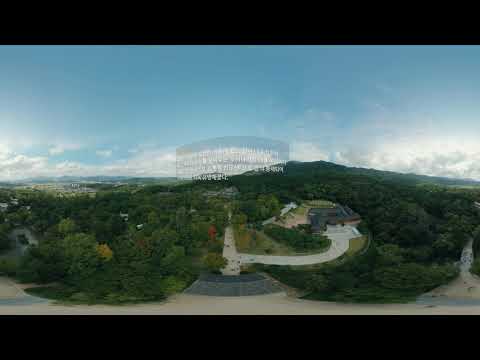This image captures a picturesque, scenic view dominated by gently rolling hills covered in dense green trees, with a few beginning to show fall colors. The sky above is a vivid blue, dotted with some wispy clouds on the horizon. Taken from a higher vantage point, the perspective gives an expansive look over a large area of land. A white concrete road runs horizontally across the bottom of the photo, leading into a paved path that veers off to the right towards a distant building, possibly on a campus or office complex. In the distance, you can glimpse a towering scaffolding structure against the sky. The image is letterboxed with long black bars at the top and bottom, suggesting it might be a still shot from a video. In the foreground, shadows and some unclear writing appear to hint at movement, perhaps a transitional frame captured in the screenshot.